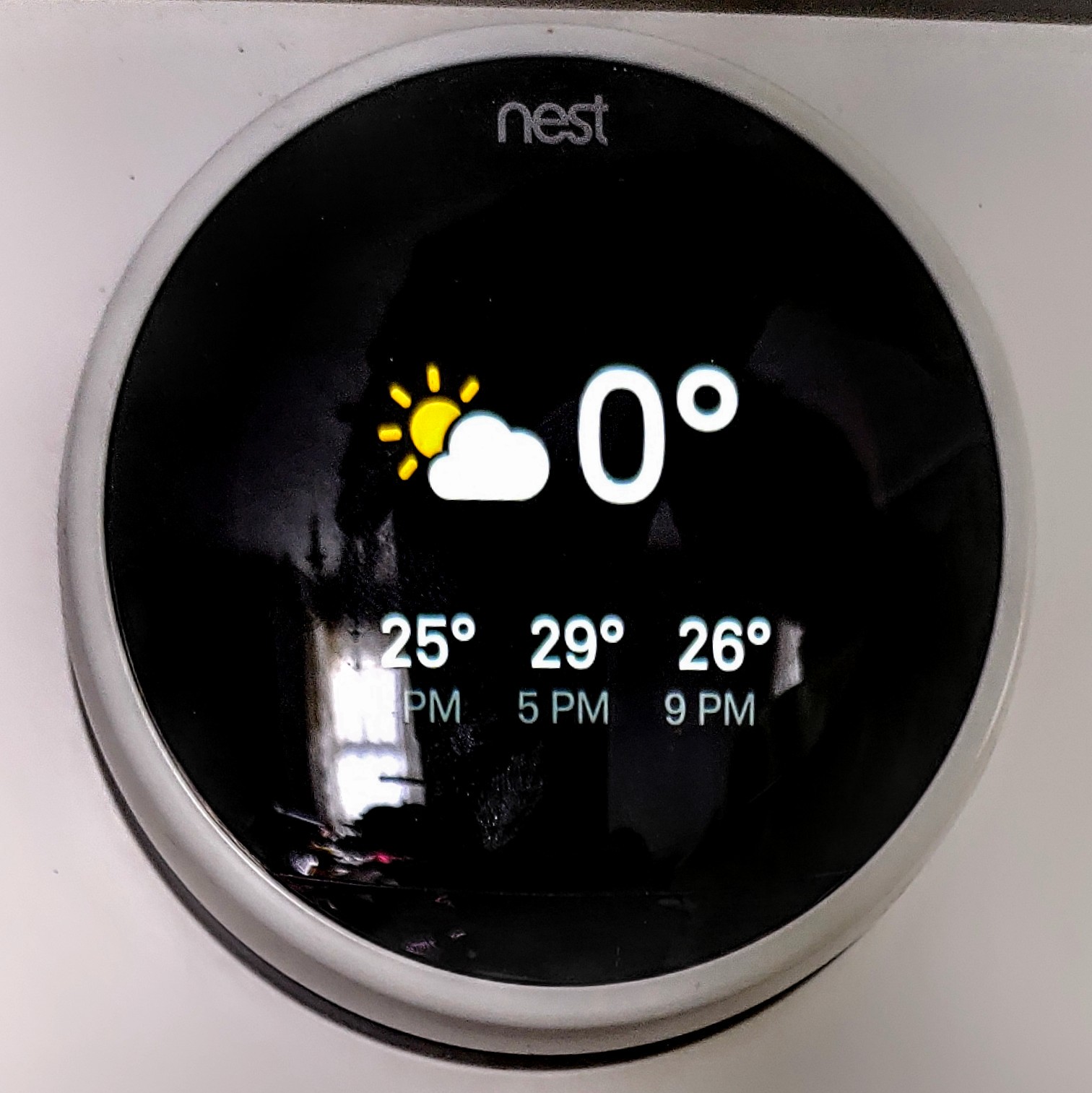The image is a slightly taller-than-wide photograph with an off-white background, suggesting it is an actual surface, likely a wall due to the slight black transition at the top. Centrally placed and nearly touching all four edges, there is a Nest thermostat. This device features an outer silver ring and a glossy black center that has a subtle bulging effect, displaying a warped reflection. The screen of the thermostat shows a partly cloudy icon and a current temperature of 0 degrees, forecasting 25 degrees at night. There is also a glimpse of subsequent temperature readings: 29 degrees at 5 p.m. and 26 degrees at 9 p.m. However, a glare partially obscures the time information. At the top of the display, the brand name "Nest" is written in gray, lowercase letters, with a distinctive 'n' that lacks the left stroke typically found in standard lowercase 'n' characters.